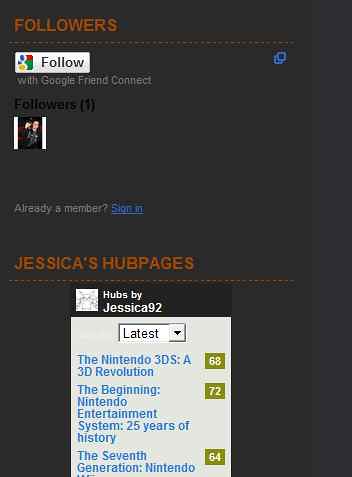The image is a screenshot of a website or an app with a predominantly black background and a dark blue vertical strip on the right side. At the top left, there's orange text that reads "Followers," followed by a Google follow icon and the phrase "Follow with Google Friend Connect." Below this section, there's a small user image under the heading "Followers (1)," and text that says, "Already a member? Sign in." Further down, also in orange text, it reads "Jessica's Hub Pages," followed by a section titled "Hubs by Jessica92." This section is sorted by the latest entries and includes clickable blue links to articles, namely "The Nintendo 3DS: A 3D Revolution" (scored 68), "The Beginning: Nintendo Entertainment System - 25 Years of History" (scored 72), and "The 7th Generation: Nintendo" (scored 64).